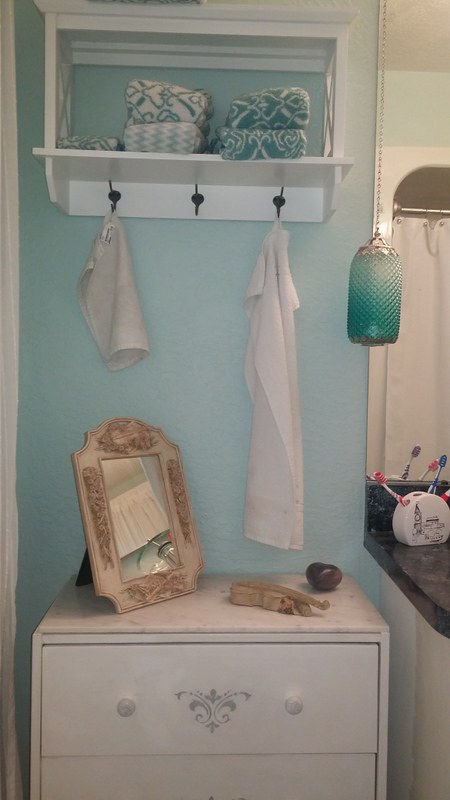This vertically oriented color photograph captures a serene bathroom scene, primarily focusing on the left side of the counter and mirror area. The backdrop is a soothing powdery light blue wall. Mounted to the upper section of the wall is a wooden towel rack holding two neatly folded towels. Below this rack, three black hooks support a washcloth and a hand towel.

At the bottom of the photograph sits a small painted white dresser, adorned with a gray design on its drawer positioned between two knobs. Atop this quaint cabinet rests an assortment of items, including a stand-up mirror and a picture frame. Adjacent to it, hanging from the side of the dark granite countertop, is a green frosted glass light, adding a touch of elegance to the space.

On the countertop itself, a toothbrush holder with three toothbrushes is prominently displayed. Reflected in the mirror, one can see a glimpse of the shower curtain in the background. The lighting in the image creates subtle shading and highlights, particularly at the top portion, enhancing the tranquil ambiance of the bathroom.